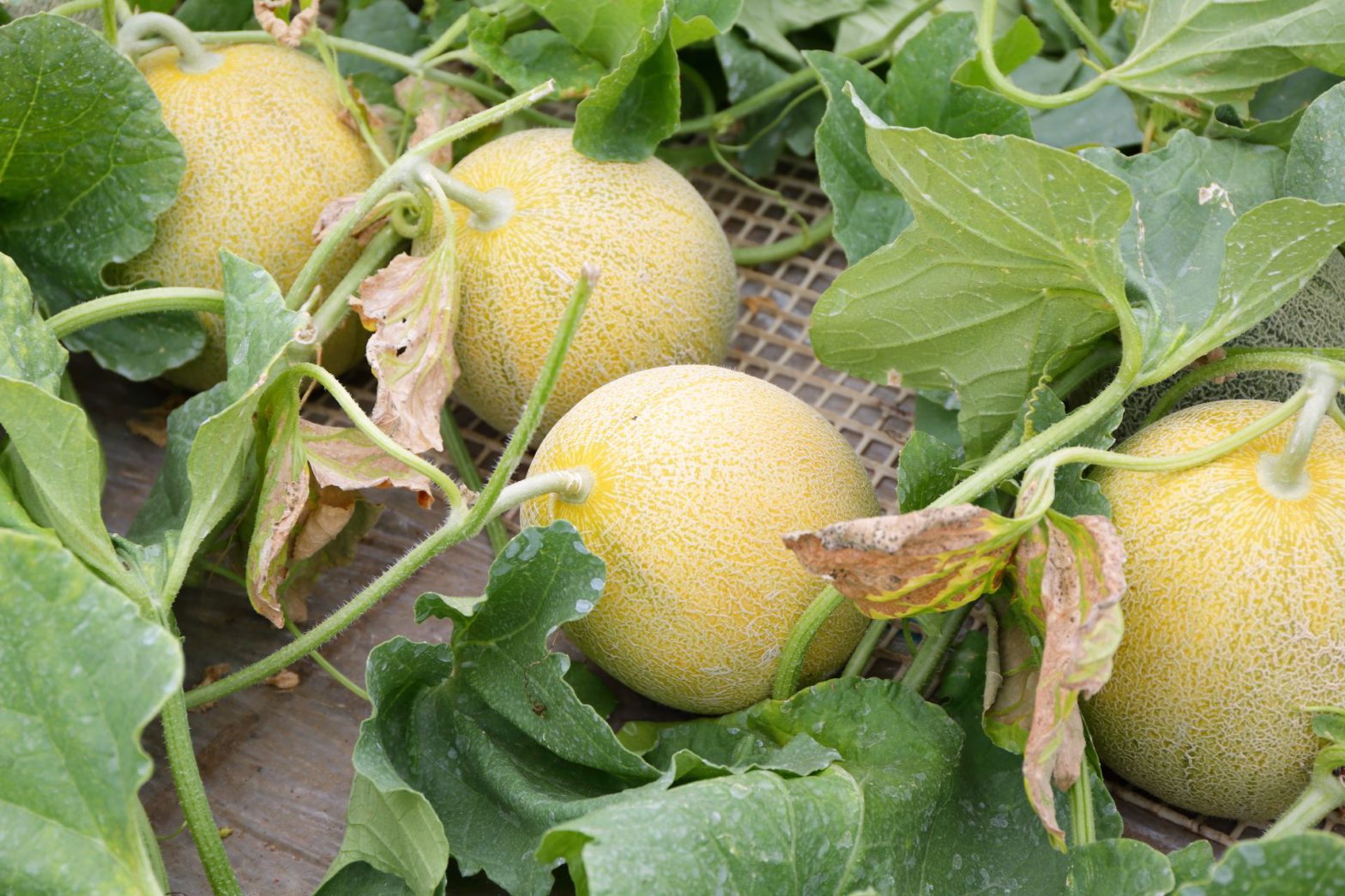This photograph captures a close-up view of four cantaloupes growing on their vines. The cantaloupes are pale greenish-yellow with a rough, cream-colored webbing texture indicative of the typical cantaloupe surface pattern. The vines and stems are fuzzy, robust, and hardy, with some curling while others stretch out. The large leaves surrounding the fruit are predominantly bright green, although some have yellowed or dried to a brown color, suggesting varying stages of health. Speckles of white on the leaves hint at possible water or calcium stains. The melons and their connecting vines are resting on an off-white mesh material, which overlays part of a wooden bench or slab, providing a structured base for the growing fruit. Overall, the cantaloupes appear nearly ripe and remarkably blemish-free.